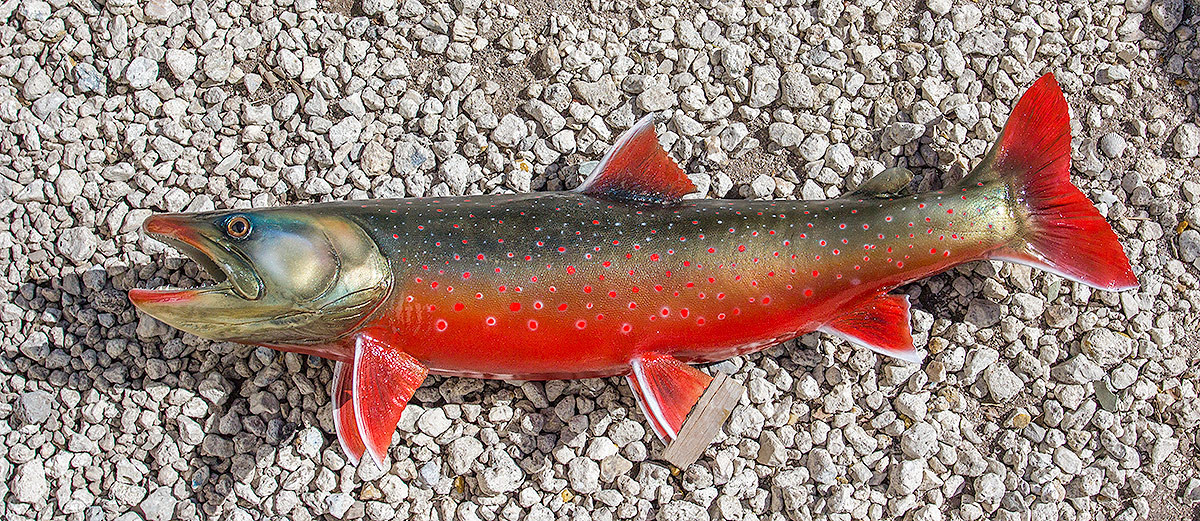The image displays a detailed photograph of a long, slender fish, likely a trout, resting on a surface of small, white gravel. The fish, distinguished by its stunning coloration, features a predominantly silver-gold body adorned with numerous vibrant red dots. Its underbelly and fins are a bright, vivid red, with five red fins on the underside and a singular red dorsal fin on top, all accented with white stripes along the edges. The fish's open mouth reveals red lips, and its eyes are marked by a striking yellow iris encircling black pupils. The fish appears freshly caught and is arranged horizontally with its body upright. The sunlight shining on the fish and gravel surface creates a sharp and almost surreal image, leaving some ambiguity about whether the fish is real or a highly detailed model.